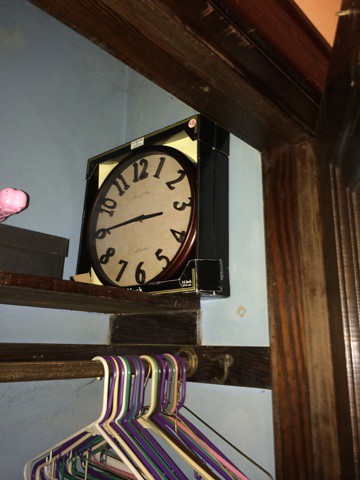The image showcases a wooden armoire or closet, characterized by its dark wood trim and an open door that reveals its interior. Inside, a square clock with a round face, seemingly made of wood, is positioned facing the side. The clock features Arabic numerals from 1 to 12, and the time indicated is approximately 3:45, with the hour hand slightly past the 3 and the minute hand pointing directly at the 9. Above a horizontal bar that spans the width of the armoire, there are several coat hangers made of both plastic and metal, clustered together on the pole. A small pink object is visible on the left shelf within the armoire. The top part of the wall above the armoire is painted a vibrant orange, adding a splash of color to the scene.